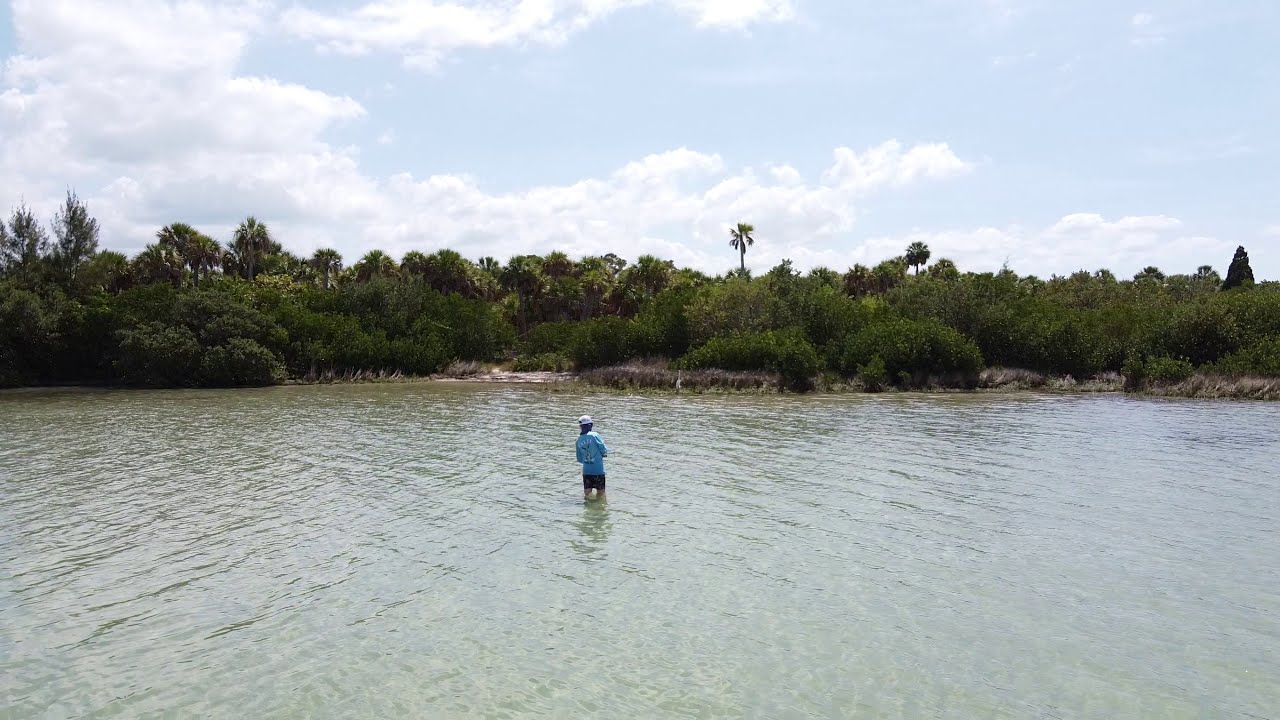The image captures a white male wearing a white cap, a light blue shirt, and dark shorts, standing in knee-deep, relatively clear water that extends across the bottom half of the photograph. The water, light-colored and reflecting the sunlight, reveals eddies and currents, hinting at a possible sandy bottom. The man is positioned centrally, facing a shoreline densely populated with various types of green vegetation, including bushes, shrubs, and trees. A single tall palm tree stands prominently against a backdrop of a partly cloudy sky, with patches of blue and sunlight filtering through. The view appears to be taken from a higher vantage point, possibly a drone, making it a landscape orientation shot. Though no fishing gear is visible, the man's stance and direction suggest he might be heading back toward the shore, where small areas of brown dirt peek through the lush greenery and small buildings are faintly visible in the distance. The sky overhead combines light blue hues with gray and white clouds, enhancing the image's bright and sunny atmosphere.